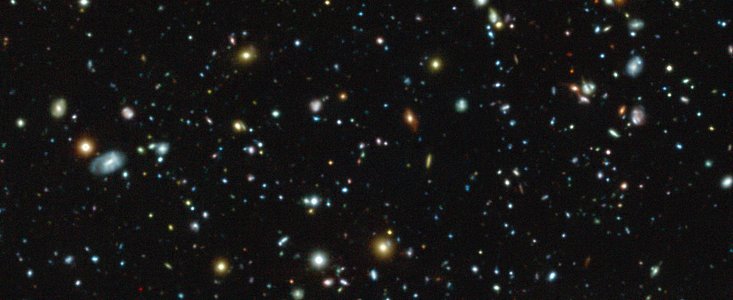This captivating photographic image depicts an expansive view of the night sky taken outdoors. The image, in a horizontal rectangular format, features a dark, nearly black background that accentuates the beauty of the celestial display. Scattered across the sky are roughly a hundred stars, predominantly clustered in the top right-hand corner. These stars vary in colors and sizes, ranging from bright oranges, whites, and yellows, to deep reds and subtle turquoise hues. Some stars appear to have a distinct halo effect, making them glow luminously against the dark canvas. Among these celestial bodies, a few objects stand out; one, in particular, has an oval shape, distinguishable from the typical spherical stars. Additionally, a prominent band of three stars can be seen right in the middle of the image. The lack of any visible constellations or text adds to the sense of infinite space, evocatively capturing the vastness and mystery of the galaxy.